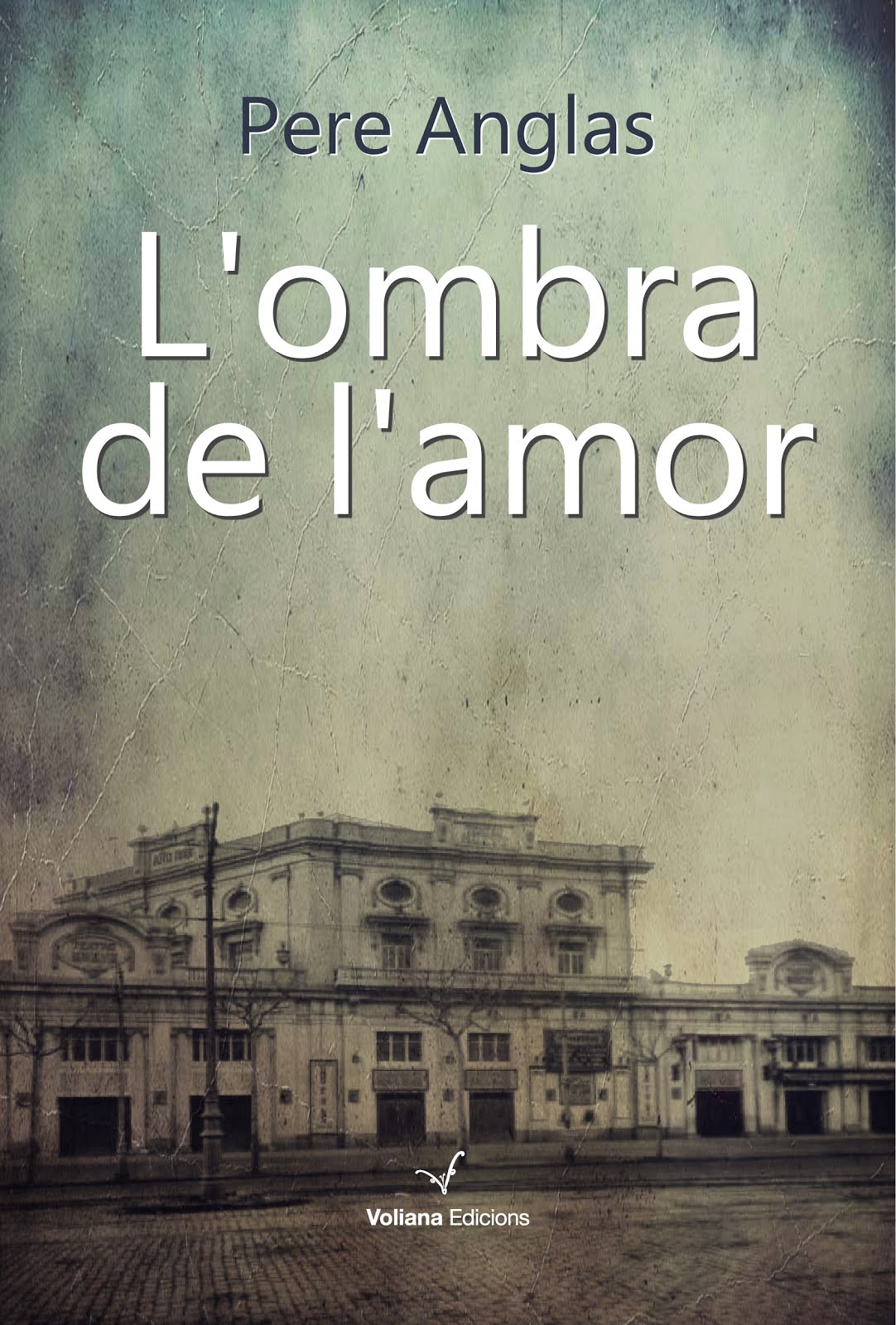The image depicts the cover of a book titled "L'Ombra de l'Amour," with text in white on a predominantly black, white, and grayscale background. The author, Pere Angelos, is listed at the top in black text. Below the title, at the bottom center, in small white text, it says "Voliana Ediciones." The background features a black and white photograph encompassing roughly 60% sky with clouds. At the bottom, a street lined with bare trees and electricity poles stretches before a prominent white, two-story building. The building’s central section is taller with various entryways and windows, flanked by shorter side sections. Additional details include a subtle street sign and a logo resembling a 'V' associated with "Voliana Ediciones." The overall composition conveys a sense of nostalgic elegance, captured in the photo and enhanced by the monochromatic color scheme with hints of off-green and off-blue.